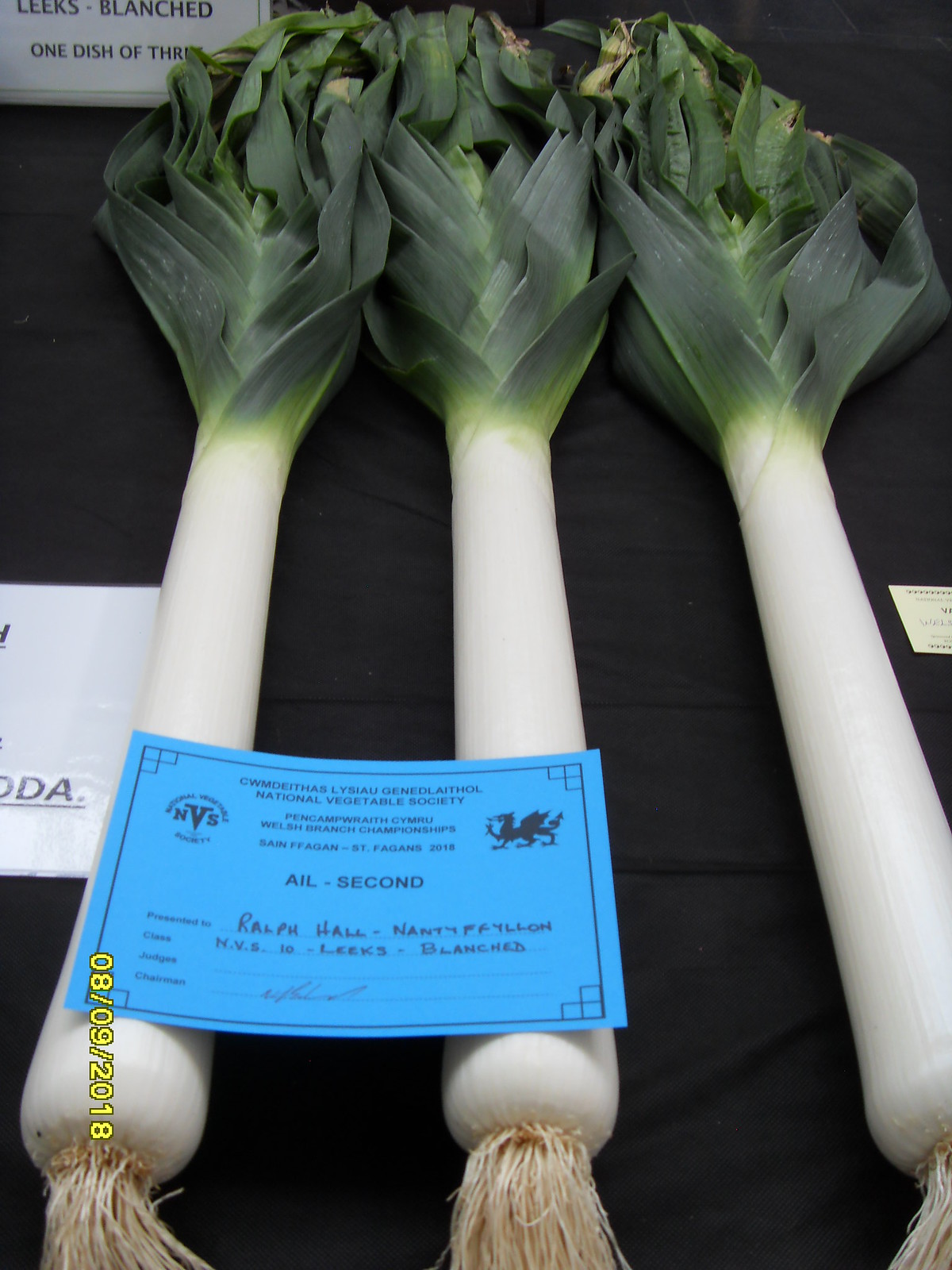This image showcases three pristine leeks arranged side by side on a black tablecloth. The leeks feature long, immaculate white stalks seamlessly transitioning into dark green, neatly trimmed leaves at the top. Draped across two of these vegetables is a vivid blue certificate. The certificate bears the heading "National Vegetable Society" and within its center, prominently reads "Ail Second," indicating a second-place accolade. It further details "Welsh Branch Championships" and includes additional text in Welsh, which appears to name the event as "Cwym Deith Lysaw Gynedlaethol." Notably, the certificate signifies the leeks' participation and victory in a vegetable competition, with the photo dated August 9, 2018. The presentation highlights the superior quality and careful cultivation of the winning leeks.